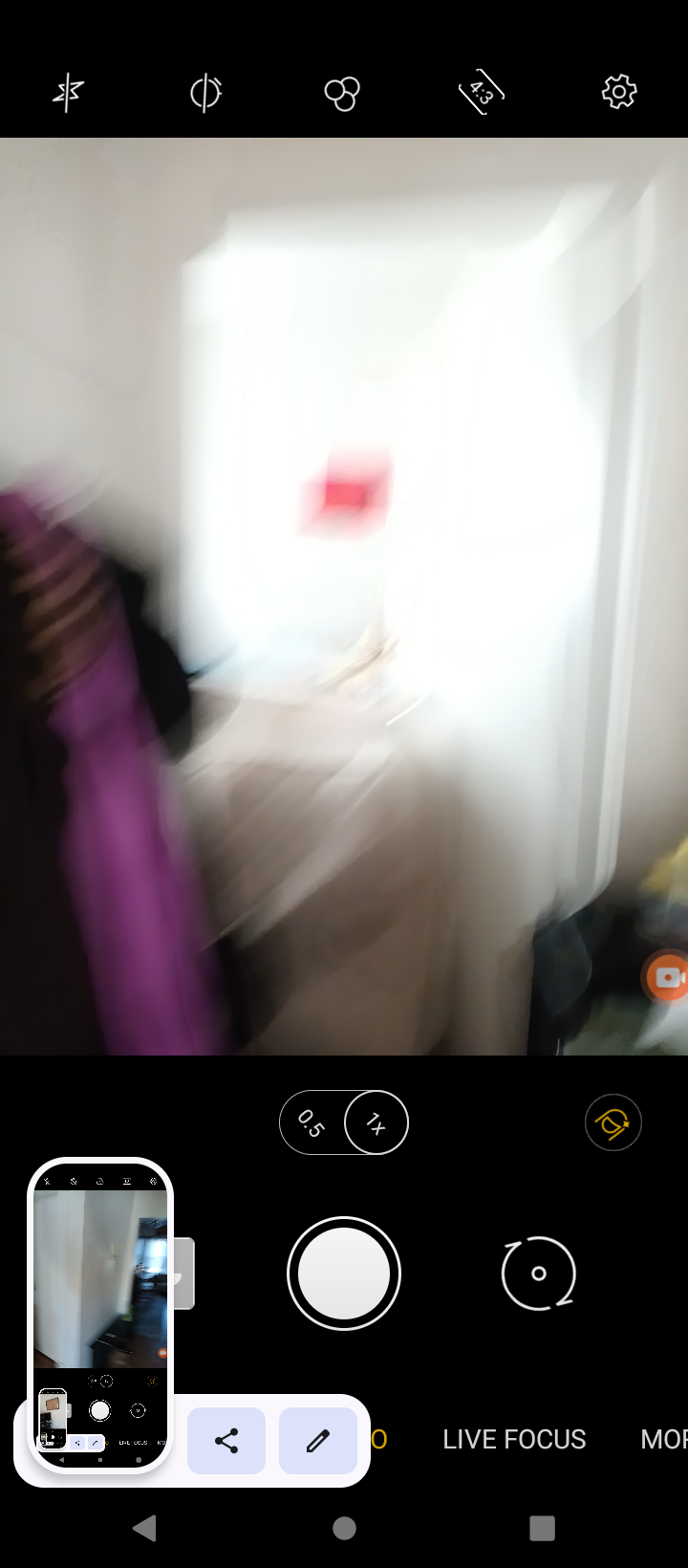This image is a highly ambiguous and blurred screenshot, possibly an accidental one, captured on a smartphone, likely an iPhone or Google Pixel. It prominently displays the camera interface, with both top and bottom bars visible. The top bar includes options for adjusting photo dimensions, applying filters, enabling flash, and accessing additional settings. The bottom bar shows magnification controls, image rotation, live focus toggles, and filter options. The background reveals an indistinct scene, possibly someone's room or a hallway with a door frame, but details are obscured due to the blurriness.

Interestingly, the bottom left corner of the screenshot contains a tiny preview of a previous screenshot, which shows yet another blurry hallway scene, creating a recursive, seemingly endless loop of screenshots. This phenomenon gives the impression of a series of random, unintentional captures, each fragmentally displaying an increasingly smaller portion of blurred images within images.